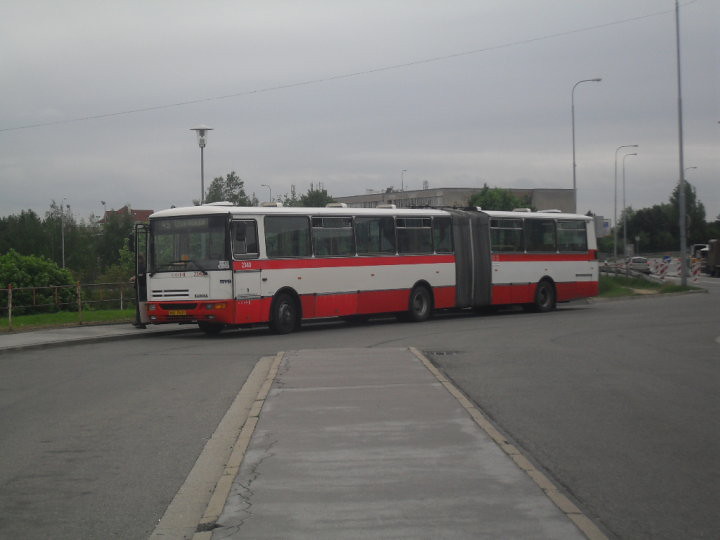The photograph captures a dreary, cloudy day with a long, articulated bus prominently displayed in the foreground. The bus features distinct white and red stripes; specifically, it has a white upper section with a horizontal red stripe below the windows and red along the lower section and around the wheels. The bus is positioned on a gray concrete street, bordered by a gray sidewalk. The articulation joint, a flexible rubber section, is visible in the middle of the bus, allowing it to bend easily around corners. In the background, several tall street lights rise into the cloudy gray sky. The scene also includes gray buildings, numerous trees, and a fence, together painting a picture of an overcast day in an urban area. The photograph is taken from a low-angle side front view, emphasizing the bus's elongated structure and the surroundings.